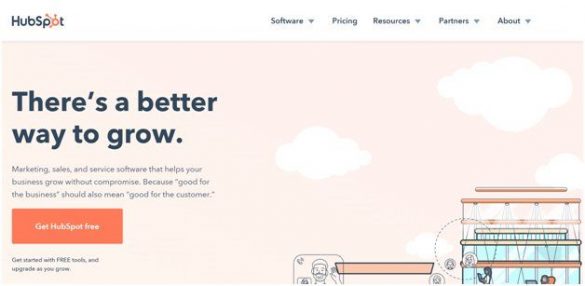The image features a top navigation bar with the HubSpot logo prominently displayed on the left. The logo is distinctive, with the "O" in orange and accented with radiating lines. To the right, the navigation options read "Software," "Pricing," "Resources," "Partners," and "About," each accompanied by a downward-pointing arrow indicating dropdown menus. The background is a soft pinkish hue adorned with wispy white clouds. Lower in the image, there's an illustration or stylized depiction of a building in orange and green tones, accompanied by various circles and an image of a man holding a camera. At the center of the image, a bold blue text states, "There's a better way to grow." Below this slogan, small black text is present, though it's too tiny to decipher. Further down, an orange rectangle contains unreadable text, and below this, there's a highlighted word "FREE" in all caps with additional illegible text surrounding it.